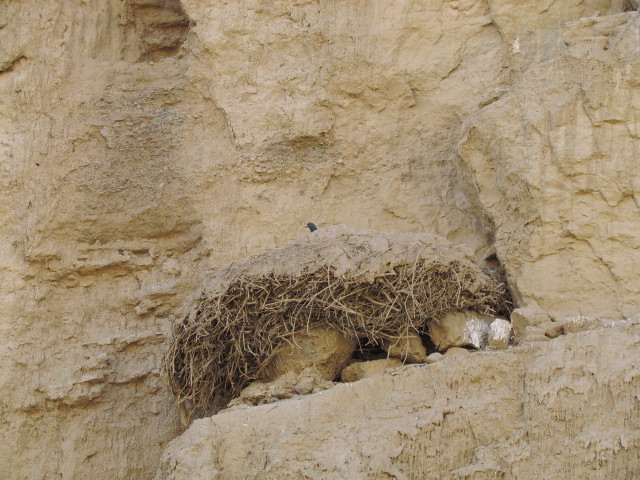This highly detailed photograph captures a sandy-colored, craggy cliff, resembling the side of a mountain or canyon wall. The cliff sports various intricate textures and is uniformly shaded, giving it a consistent beige tone devoid of direct sunlight. In the top left corner of the image, there appears to be a small cave opening or natural hole. The bottom center prominently features a ledge consisting of several large rocks upon which rests a sizable nest. This nest is loosely constructed from twigs and dry reeds, with the top covered in a layer of mud or sandy material, securing the structure. The nest is home to a very small pigeon, whose gray head is just visible above the nest’s rim. Additionally, there is some buildup resembling tumbleweed or hay around the nest. The overall composition of the photo, taken from a slightly upward angle, emphasizes the quaint sanctuary embedded within the vast, rugged expanse of the cliff.